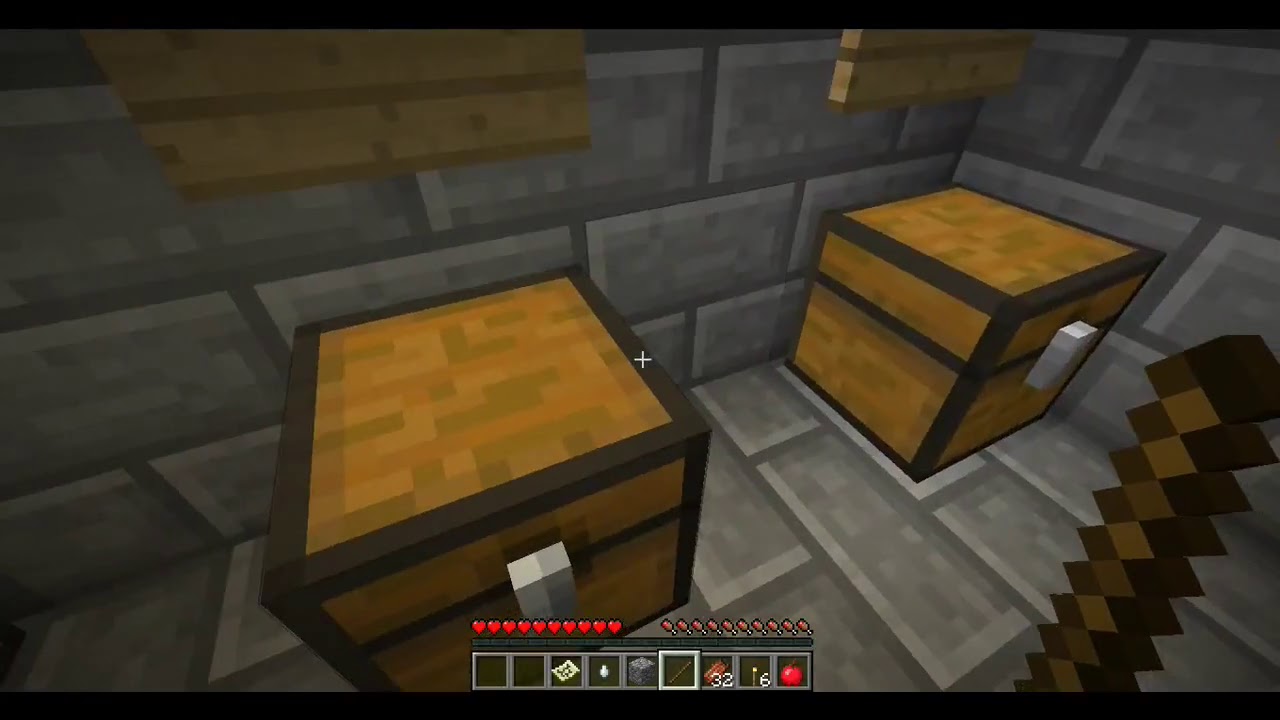This is a horizontal, pixelated image that appears to be a screenshot from a computer game, reminiscent of Minecraft. The scene is set in what looks like a dungeon or castle, constructed from gray stone bricks that cover both the floor and walls. In the foreground, there are two square, wooden chests with dark brown trim and possible locks on the front, positioned on a tiled floor. The one on the right is nestled in the corner of the room, while the second chest is a short distance away from the first. 

In the lower right corner, there is an additional object with spikes, though it's too indistinct to identify clearly. Across the bottom of the screen are various clickable icons, including minute hearts likely representing lives, and small boxes containing items such as a red apple, a ticket, and a candle. The bottom border also displays numbers like 32 and 6, possibly indicating scores or quantities of items. The image is framed with black borders on the top and bottom, adding to the overall dark ambiance.